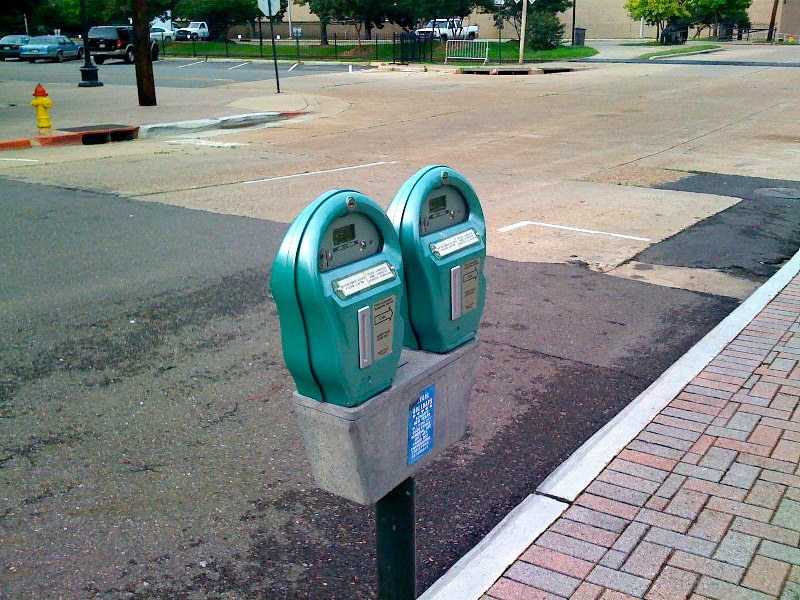This photograph depicts a parking lot in an American town, with an emphasis on a prominent parking meter and various background details. Central to the image is a pair of bright turquoise parking meters mounted on a single black pole with a blue, slightly peeled sticker. Each meter features a coin slot, time display, and accepts only coins, indicating spaces for two vehicles. The pole is rooted in a decorative brick sidewalk, composed of various shades of red and brown stones.

In the background, a faded, slapdash-repaired street extends with clearly painted parking lines, suggesting a well-used urban area. Across this street sits a distinct yellow fire hydrant topped with a red cap, which is easily visible. Surrounding the hydrant and parking meters are several parked vehicles, including a black truck, a baby blue sedan, and a white SUV, among others. A diverse array of elements like trees with dark brown trunks, green grass, and low bushes bring a touch of nature to the otherwise urban scene. Additional structural features such as a lamppost, a stop sign, a fence, and the façade of a distant building are also noticeable, but the parking meter and the hydrant dominate the composition.